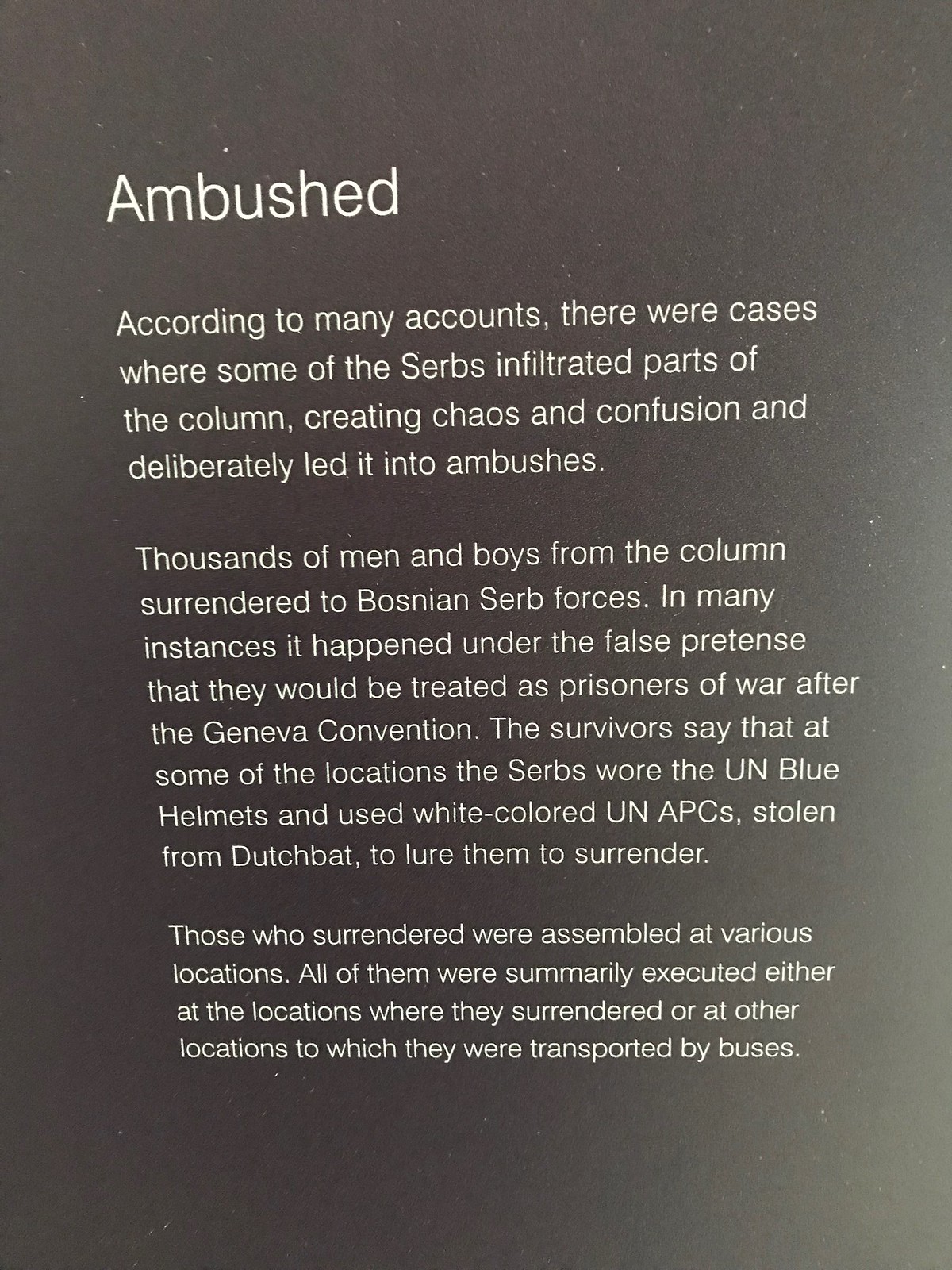The image is a vertically oriented rectangular panel, appearing to be part of an exhibit, possibly next to a photographic display. It features a dark gray, almost black background with stark white text, giving it a solemn, authoritative presence.

At the top, prominently left-aligned, the title "Ambushed" is displayed in bold white letters. Beneath it, three paragraphs of left-aligned text provide a harrowing account:

1. "According to many accounts, there were cases where some of the Serbs infiltrated parts of the column, creating chaos and confusion, and deliberately led it into ambushes."
2. "Thousands of men and boys from the column surrendered to Bosnian Serb forces. In many instances, it happened under the false pretense that they would be treated as prisoners of war according to the Geneva Convention. Survivors recount that at some locations, the Serbs deceived them by wearing UN blue helmets and using white-colored UN APCs stolen from Dutchbat."
3. "Those who surrendered were assembled at various locations. All of them were summarily executed, either at the surrender sites or at other locations to which they were transported by buses."

The text effectively conveys the tragic events, emphasizing the deception and subsequent atrocities committed during the conflict.